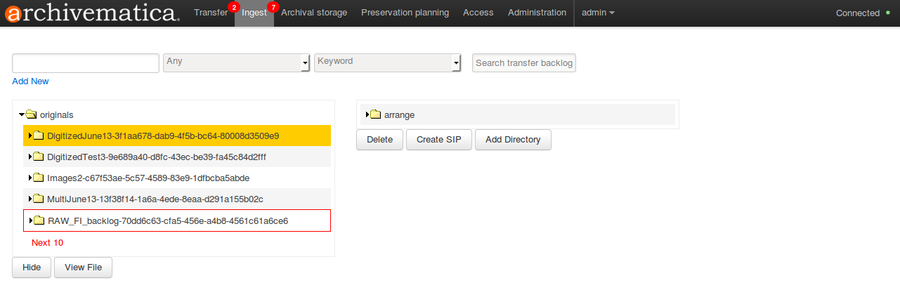This colorful landscape screenshot captures the interface of a user's session on Archivematica, a digital preservation software. The interface is simple and functional, designed more for utility than aesthetics, with the main navigation tabs displayed prominently on a black banner at the top of the screen. These tabs, written in lowercase white letters, include: Transfer, Ingest, Archival Storage, Preservation Planning, Access, Administration, and Admin. The only exception to this monochromatic scheme is the ‘is’ within the word 'Administration' which overlaps with an orange circle, standing out visually.

On the top right corner, a green circle indicates the system's ‘Connected’ status, ensuring the user of their current connectivity. Below the main banner, the interface offers several interactive options such as "Add New," along with dropdown menus for selecting any specific options or keywords, and a "Search Transfer Backlog" function for efficient file navigation.

The main content area displays a structured view of folders and subfolders, beginning with an 'Originals' folder which branches out into various other folders labeled as 'Digitized June 13th,' 'Digitized Test 3,' 'Images 2,' and 'Multi-June.' These folders likely contain different sets of digitized documents or images that the user can hide, view, or delete as necessary, making the management of archival materials straightforward and organized.